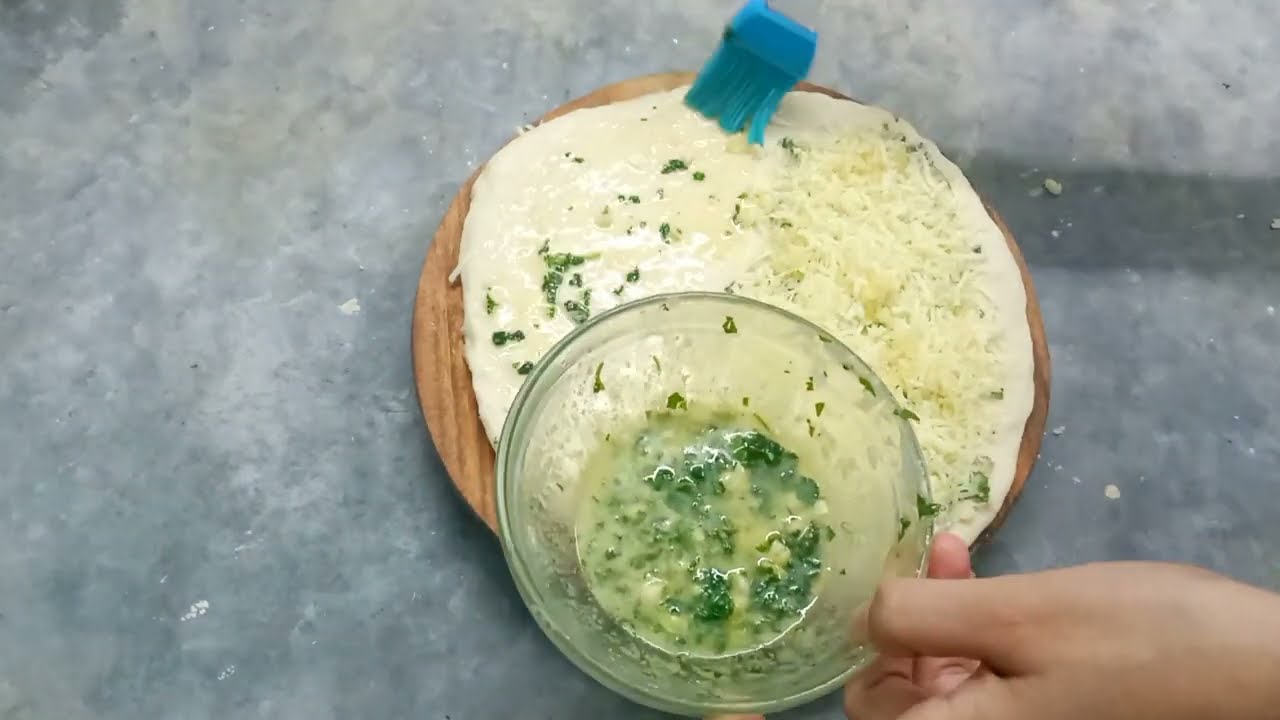In this image, taken from an overhead perspective, a tortilla rests on a round wooden board that resembles a Lazy Susan, precisely matching the tortilla in size. The scene is set against a dark gray, mottled marble countertop which serves as the background. The tortilla itself is partially covered with white shredded cheese on the right-hand side. On the left side, a small glass bowl containing a green, herb-infused butter or oil mixture is being held by someone with their left hand. This hand appears towards the bottom of the image. They are using a silicone basting brush with a blue tip and a clear handle to apply the mixture onto the tortilla. The blue brush tip is clearly visible at the top of the screen, showcasing the spread of this liquid mixture over the left half of the tortilla.